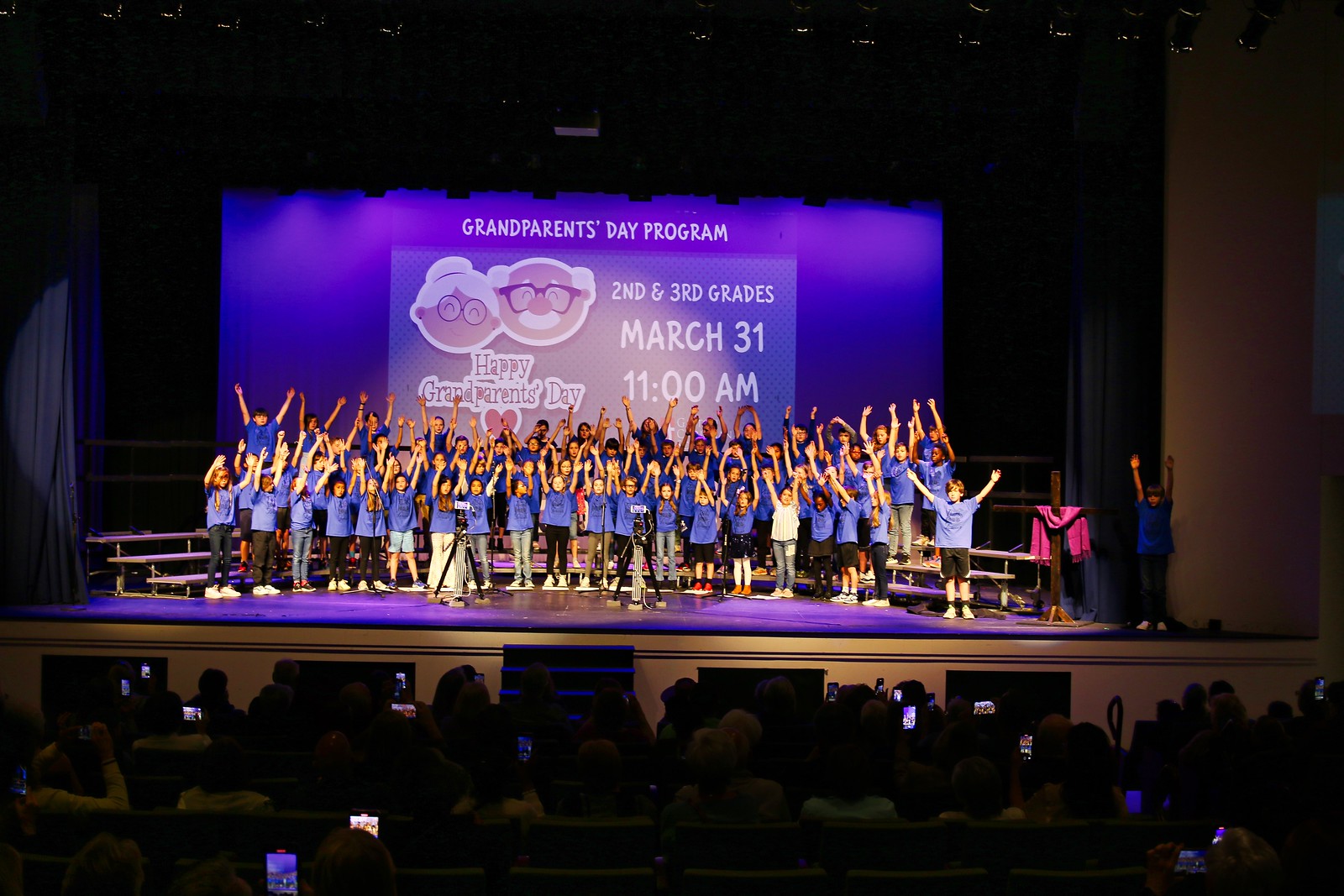Inside a spacious auditorium, a vibrant Grandparents Day Program unfolds on March 31st at 11 a.m. The stage is brimming with lively energy, occupied by around 40 children, likely second and third graders, standing on risers in three neat rows. Most of the children are dressed in blue T-shirts paired with either black or blue bottoms, including jeans, shorts, and pants, though one notably stands out in a white T-shirt. All of them have their hands enthusiastically raised in the air, as if concluding their performance with a grand finale.

Behind the children, a large blue screen displays cheerful, cartoonish depictions of a grandmother with white hair and a grandfather with a white mustache, beneath the heading "Grandparents Day Program." Alongside, the text announces, "Second and Third Grades, March 31, 11 a.m." A cross draped with a pink cloth can be seen to the right of the children, adding a touch of solemnity to the scene.

In the foreground, we catch glimpses of the audience, their attention fully captivated by the children's performance, while a few attendees hold up cameras to capture the memorable moments. The festive atmosphere is palpable, with the interplay of youthful exuberance and heartfelt celebration honoring grandparents.